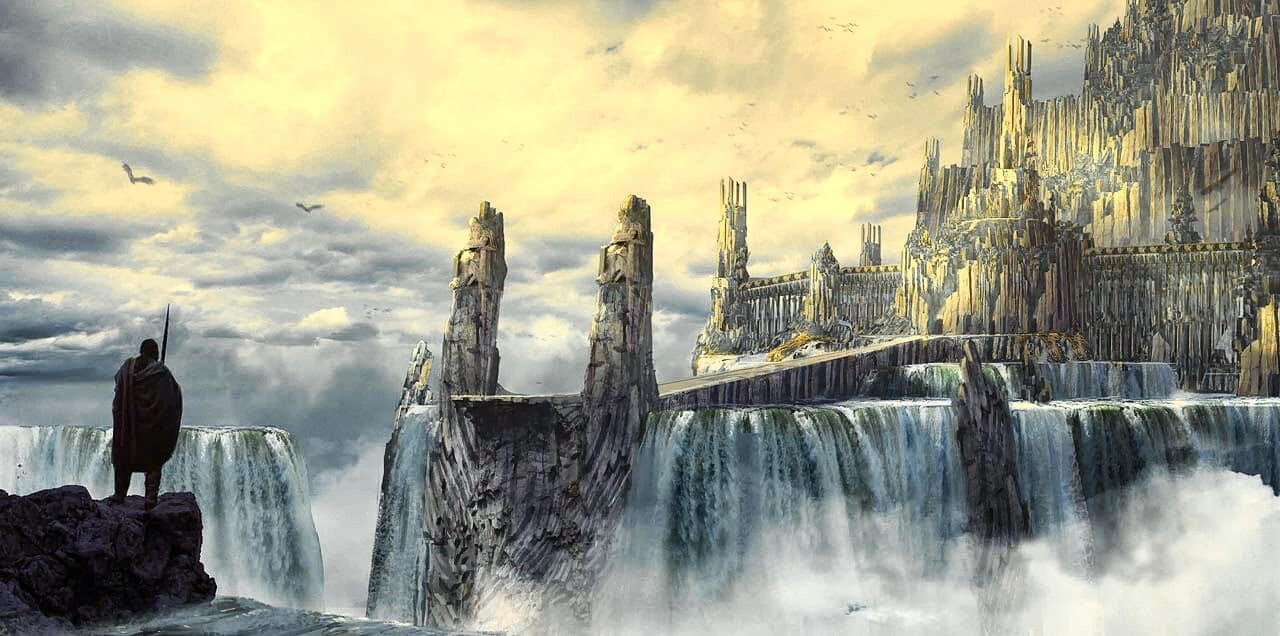In this captivating daytime scene, reminiscent of a fantasy realm akin to Lord of the Rings, we see an elaborate and imposing castle formation dominating the right side of the artwork. This castle, seemingly sculpted from dark granite-like rock in hues of grays, blacks, yellows, and creams, rises majestically with tall, spiny features that converge into its towering walls. The structure brims with multiple layers, broader at the base and narrowing as they ascend, adorned with high turrets crowned by jagged teeth-like spires. From the base of the castle, powerful waterfalls cascade down in torrents, creating misty puffs as they crash into the waters below, adding to the ethereal ambiance. 

The backdrop is a cloudy sky, sporadically dotted with birds that add a sense of scale and freedom to the otherwise towering and looming castle. Bridging the castle to the foreground is a mighty cliff that supports a bridge leading up to the castle entrance. To the left of this cliff, in the foreground, stands a solitary figure. Clad in tight leggings and a cloak wrapped around them like a blanket, the figure grips a tall spear or sword, staring into the void that separates them from the magnificent castle. The entire composition, perhaps digitally crafted to echo the feel of an artist's oil painting, evokes an otherworldly and mysterious vibe, perfectly encapsulating a realm filled with wonder and peril.